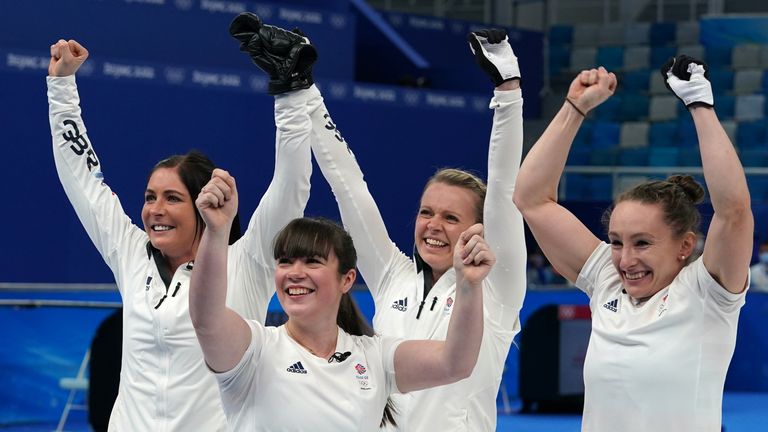The image captures a triumphant moment of four women, who appear to have just achieved a victory in a curling match at the Winter Olympics. They're all wearing white shirts with a team logo on the left side, showing a mix of long-sleeve and short-sleeve tops. Each woman is wearing a glove on one hand – two have smaller gloves that are white on the palms and black on the outside, while the other two are donning thicker, all-black gloves. The tallest woman on the left has straight black hair and stands adjacent to a woman with light brown hair, who is second tallest. The woman with light brown hair has her left fist clenched and is smiling broadly. Next, on the right, is a short woman with black hair and bangs, who is wearing short sleeves. The fourth woman has blonde hair and both hands raised, with a microphone clipped to her collar. Their arms are all raised in triumph, forming a “V” for victory. Behind them, a blur of a blue mat and a dark blurred background accentuates their victorious pose.